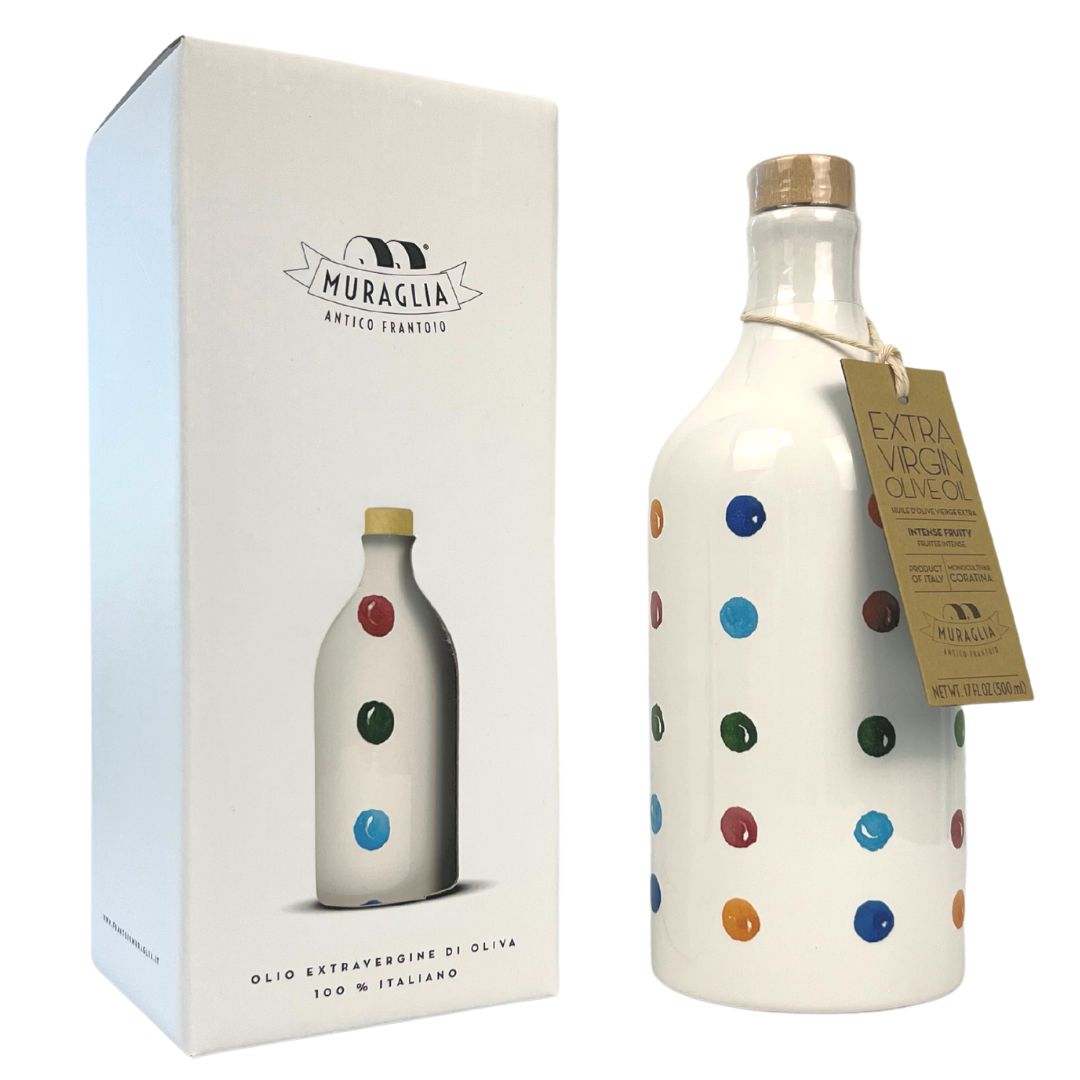In the image, we see a sophisticated bottle of Meraglia Antico Frantoio Extra Virgin Olive Oil positioned to the right, with its packaging box on the left. The scene is set against an all-white background, emphasizing the clean, elegant design. The bottle itself is primarily white, adorned with rows of colorful polka dots in dark blue, turquoise blue, green, red, pink, and shades of orange or yellow. The dots are arranged in a pattern of five rows, extending from the neck to the bottom of the bottle. The bottle features a brown cork and a matching brown label attached with a tan twine around the neck, which reads "Extra Virgin Olive Oil" along with some other less legible text. The packaging box mirrors the bottle’s design with polka-dot artwork and contains additional text in black, which includes the phrases "Meraglia", "Antico Frantoio", "Olea Extravaganza", and "100% Italiano". Both the bottle and the box present a unified and aesthetically pleasing appearance, making the product visually appealing and indicative of high quality.